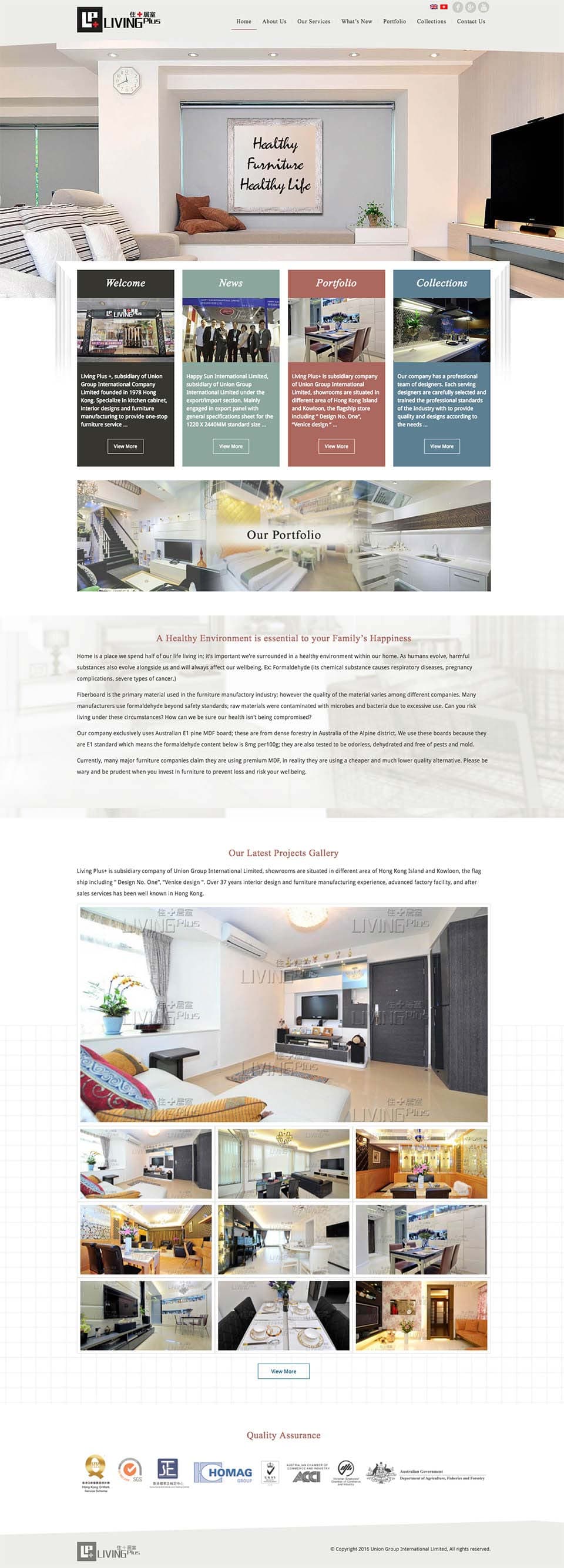Screenshot of a neatly organized webpage showcasing a home from different angles. The page features a black rectangular banner with green, red, and blue accents, containing the title "Our Practice" and detailed information about the home. 

In the main image, the room appears to be an office or living area with a comfortable ambiance. It has two large windows that let in ample natural light, a clock mounted on the wall, a dresser with a flat-screen TV, and a sofa. The layout seems cozy and functional.

Beneath the main image, there are four sections, each with pictures and additional information. The featured images show various perspectives of the same home. One image highlights the living room with windows opened, giving a fresh, airy feel. The third picture showcases a modern kitchen, while the sixth picture reveals a neatly arranged dining area with a small square table and two chairs.

At the bottom of the page, there are several logos, and the footer is designed in a subtle gray hue, adding to the overall sleek and professional look of the webpage.